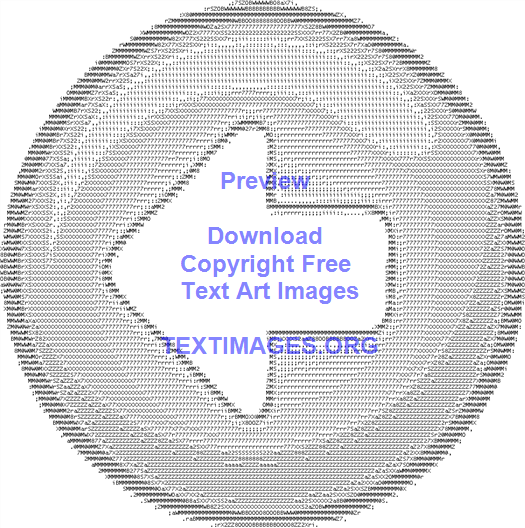The image showcases a digitally rendered, pixelated gray circle with nuanced details that blend both modern and retro aesthetics. The circle is primarily composed of intricate patterns of black text on a white background, varying in density and spacing. The outer rim of the circle features a narrower band of densely grouped text, while the inner design stretches out with more widely spaced text. At the core of the image is a conspicuous white left-pointing arrow, formed by tightly packed text outlining its shape, leaving the arrow itself as a white space. Superimposed over this arrow in light blue text are the words "Preview," "Download," "Copyright Free," "Text Art Images," and "TextImages.org," sequentially stacked. The entire circle is surrounded by an alternating blue and white border, adding to the vintage effect. Additionally, a white semicircle sits at the top, while a black and white semicircle spans from the lower center to the upper right, blending into the black and white dots scattered across the remaining background. The overall design is reminiscent of 90s digital graphics, possibly created for an early HTML website, evoking a nostalgic, old-fashioned Photoshop aesthetic.